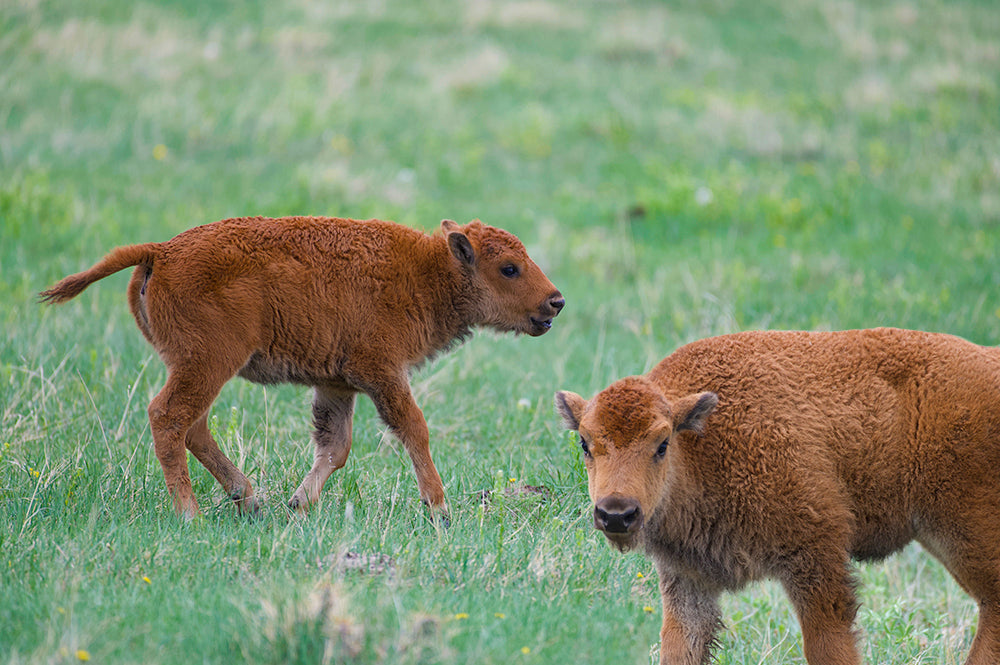The image captures a serene scene of two baby calves standing in a lush green field. The foreground of the grassy field is in sharp focus, while the background gradually blurs into the distance. Both calves have a puffy, fur coat resembling sheep's wool, but they are undeniably cows. The calf in the lower right-hand corner is facing the camera with its head turned toward the lens, revealing a black nose and perky ears. Its body is oriented to the left, and it has a notably short tail. The second calf, positioned more towards the left side and slightly further back in the image, faces straight ahead with its right side visible to the camera. Both calves are brown and appear to be very young. The overall focus on the calves and the detailed texture of the foreground grass create a vivid and endearing portrait of these young animals in their natural environment.